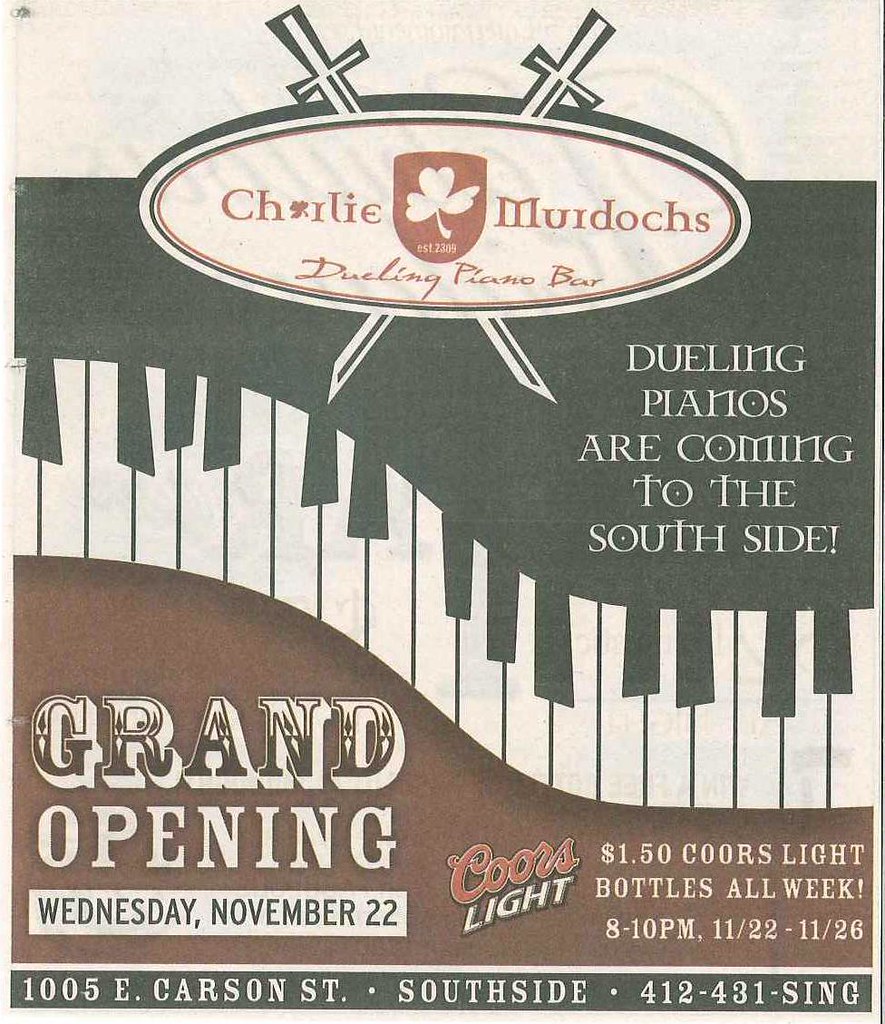The advertisement for the grand opening of Charlie Murdoch's Dueling Piano Bar sets an inviting tone with its rich Irish-themed colors of green, brown, and white. Central to the design is an oval emblem featuring the bar's name, "Charlie Murdoch's," accompanied by a brown shield and a white shamrock, along with the establishment year "Est. 2309." Two white swords with green outlines cross behind the oval, adding a touch of elegance and vibrancy that aligns with the Irish pub ambiance. The phrase "Dueling Pianos are coming to the South Side" is prominently displayed in a distinctive font reminiscent of traditional Irish typography. A unique wavy pattern of piano keys extends across the middle of the advertisement, enhancing the musical theme. The event's details stand out clearly: "Grand Opening, Wednesday, November 22," sponsored by Coors Light with a special promotion of $1.50 Coors Light bottles all week, from 8 to 10 p.m., running from November 22 to November 26. The venue’s exact location, "1005 E. Carson Street, South Side," and contact number "412-431-" ensure that potential attendees have all the information they need to join the festivities.